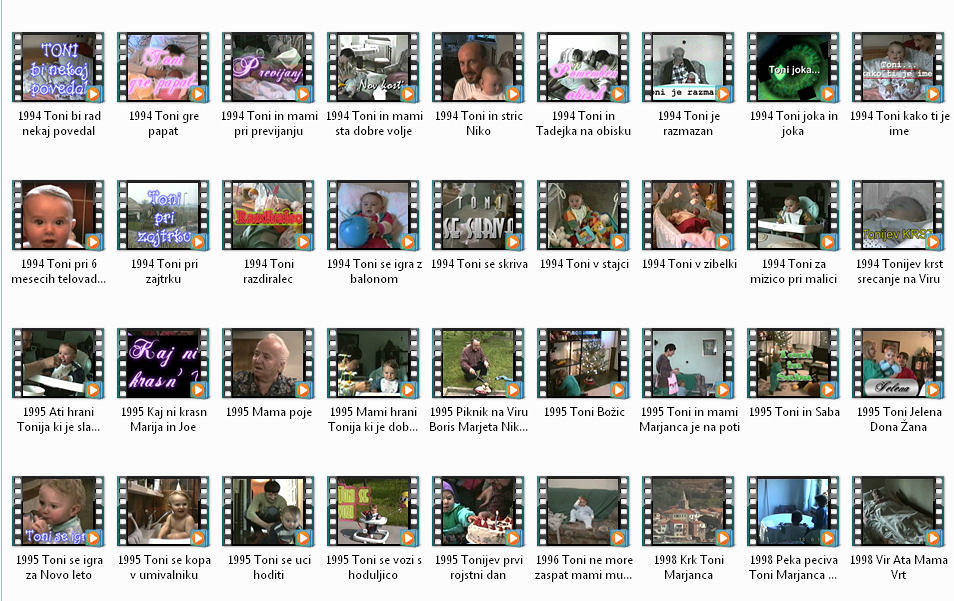The image is a screenshot of a computer folder, resembling a basic Windows file directory, with a white background showcasing 36 video files arranged in 4 rows of 9 each. Each video file is represented by a thumbnail accompanied by a film strip border and the recognizable orange-and-white Windows Media Player play button at the bottom right corner. Beneath each thumbnail, the video files are named in black text, resembling a typical Windows display, with titles beginning with dates ranging from 1994 to 1998. The thumbnails feature scenes mostly of people in various indoors and outdoors settings, suggesting these videos document different stages of life. Notably, the videos appear to be home recordings, likely converted from VHS or an older format to a digital one, given the years indicated. There are recurring subjects, including a child and an older man, with one video showing the child being held by a man who is presumably the father. The filenames and partially visible details suggest the text might be in a non-English language.